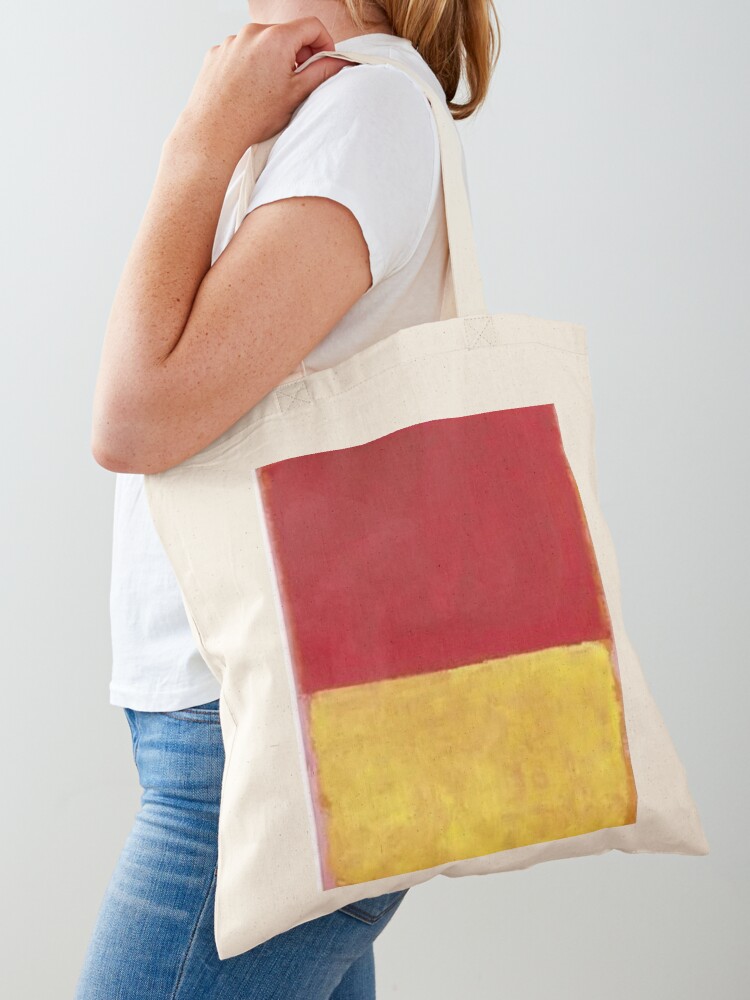A woman with fair skin and freckles on her left arm is standing against a white background, wearing a white t-shirt and blue jeans. Her dark blonde hair cascades down her back, though her face is not visible in the image. She holds a large off-white canvas tote bag over her left shoulder with her left hand. The bag features a distinctive design: a large rectangle with its top portion painted red and its bottom portion painted yellow, giving it a domino-like appearance without the dots. The painted sections fade slightly into brown around the edges and have a somewhat uneven, hand-painted look, with the yellow area showing slight dirt markings. The woman is positioned in the middle of the frame, facing slightly to the left.